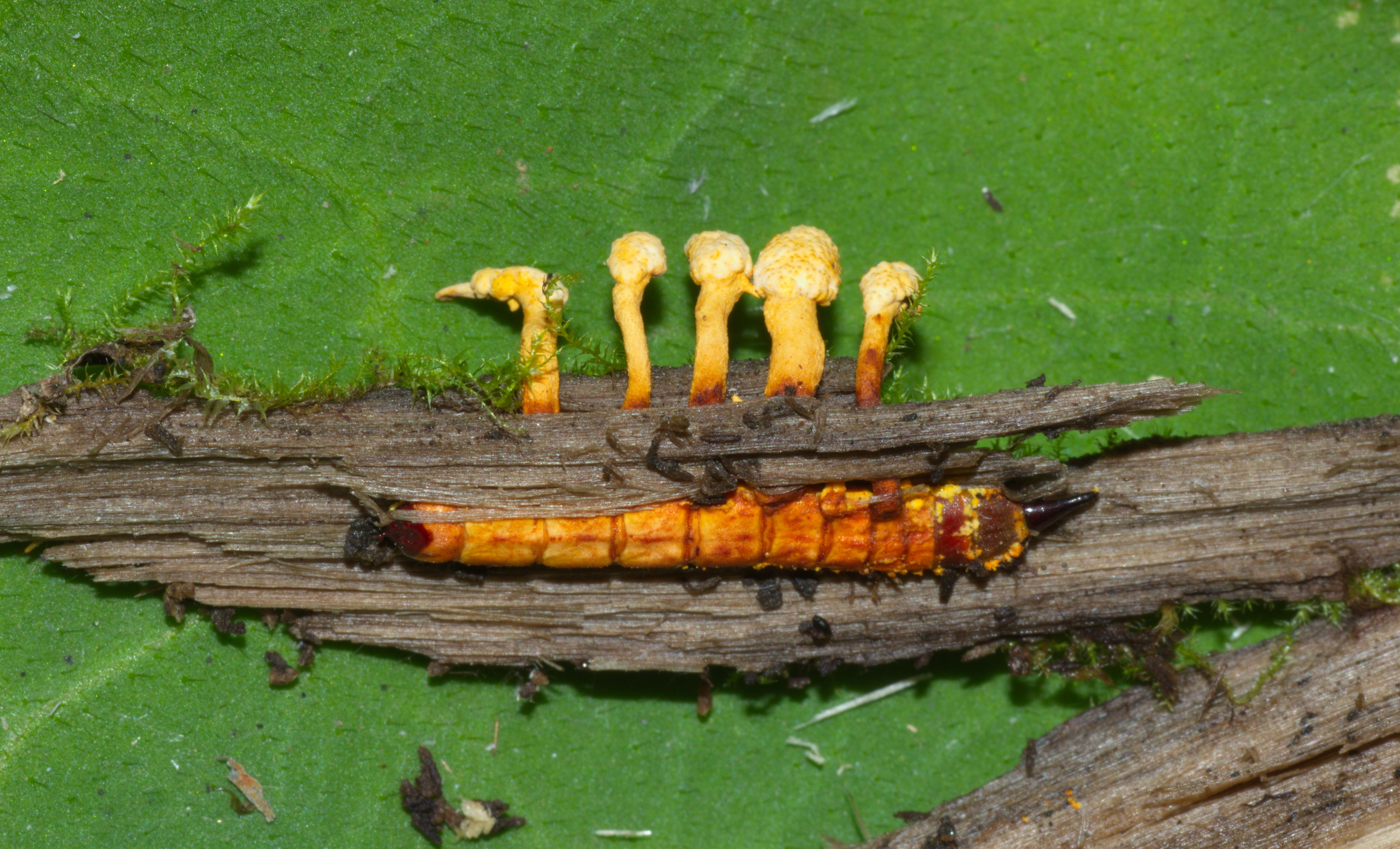A large, horizontally-placed piece of tree bark rests on a green felt background, resembling astroturf. The bark, primarily in lighter shades of brown, is adorned with small stringy pieces of moss at either end. Prominently, five elongated fungi sprout from the top center of the bark. At the heart of the bark, a striking insect draws attention; it features a burnt orange and red segmented body, culminating in a cone-shaped black tip on one end. The insect appears to have extremities or claws emerging from beneath the bark. Smaller scattered pieces accompany the main bark on the green felt, adding to the eerie yet intriguing composition of the scene.